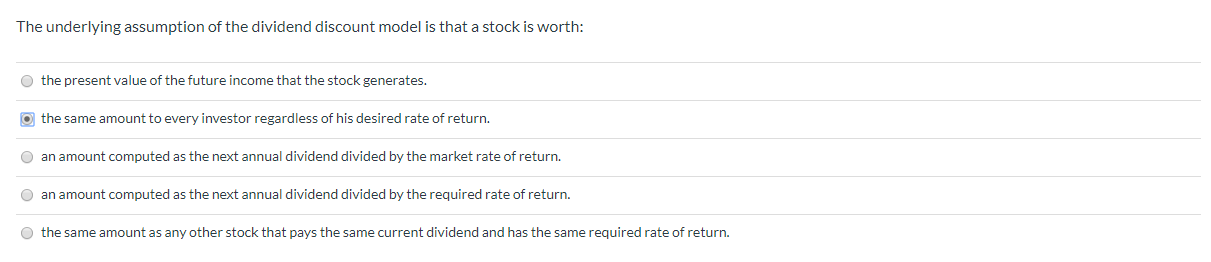This is a cropped screenshot depicting a selection of answers from a website, displayed on a white background. At the top left, medium-sized black text reads: "The underlying assumption of the dividend discount model is that a stock is worth:". Following a line break, a series of answer choices appears, each separated by thin, light gray lines that almost span the entire width of the image, leaving slight margins on the left and right. 

Each answer choice is accompanied by a circular radio button on the left, resembling a light gray orb. The second radio button is filled with a dark gray dot and is outlined by a blue square, indicating it is the selected choice. 

To the right of each radio button, black text provides different answer options. From top to bottom, the text reads:
1. "The present value of the future income that the stock generates."
2. "The same amount to every investor, regardless of his desired rate of return."
3. "An amount computed as the next annual dividend, divided by the market rate of return."
4. "An amount computed as the next annual dividend, divided by the required rate of return."
5. "The same amount as any other stock that pays the same current dividend and has the same required rate of return."

Notably, the thin, light gray line is absent beneath the final option, creating a more substantial negative space beneath the last selection in the list.